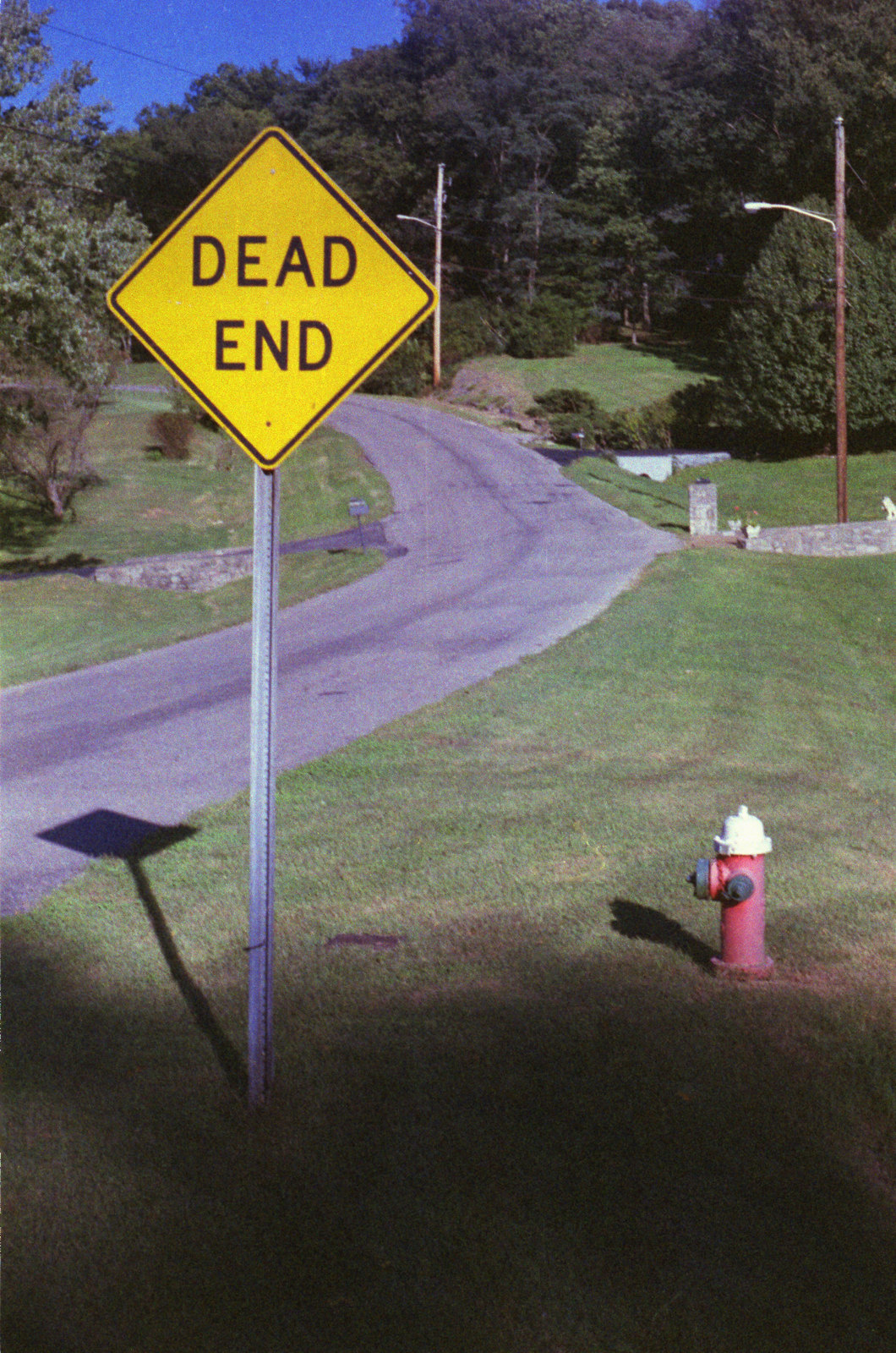In this neighborhood scene, a vivid yellow diamond-shaped "Dead End" sign with bold black lettering and trim stands prominently on a curved road, affixed to a sturdy metal pole. The well-manicured grass surrounding the area highlights the care taken in this residential community. A vibrant red fire hydrant, topped with white and featuring two black knobs for fire department use, is positioned nearby, adding a touch of practicality to the picturesque setting.

Further down the block, streetlights are suspended from telephone wires, casting future illumination on the otherwise sunny day. Majestic, mature evergreen trees line the street, providing natural beauty and shade. A meticulously crafted stone wall can be seen next to one of the houses, with another matching wall situated across the street. The road itself gently declines before curving slightly upward to the left, creating a subtle serpentine effect.

The clear blue sky overhead is entirely devoid of clouds, completing this idyllic suburban tableau.